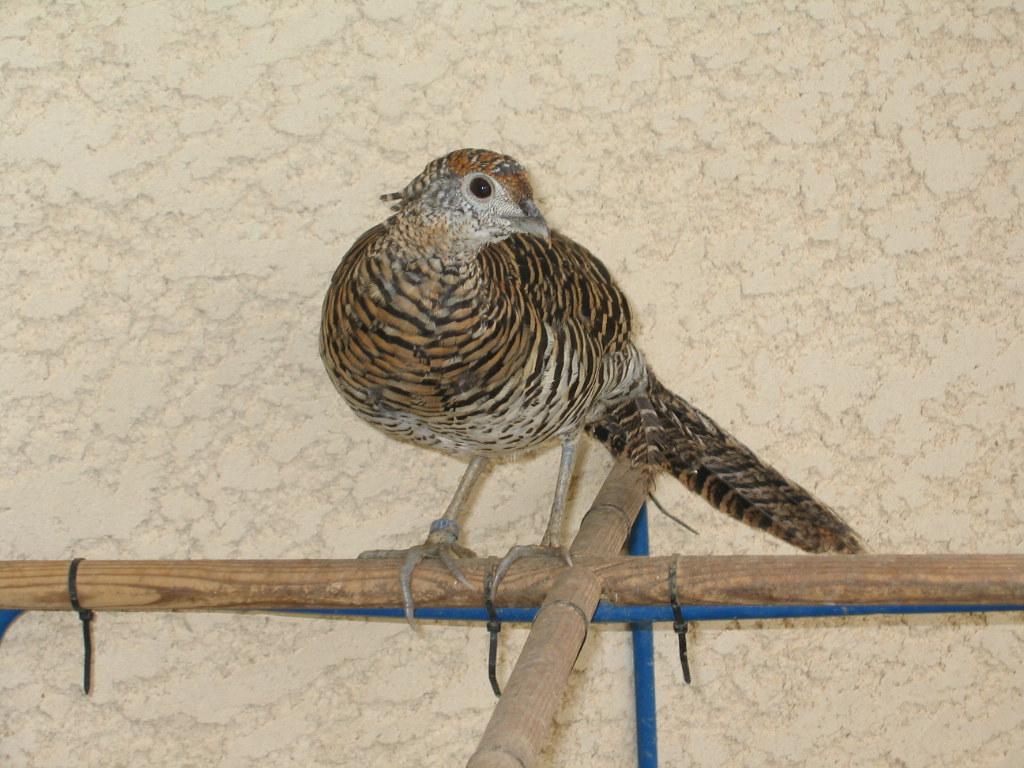This detailed photograph captures a medium-sized bird perched on a T-shaped dowel, zip-tied to a metal framework for stability. The bird showcases a striking combination of black, tan, and white feathers, with a distinctive pattern reminiscent of tiger stripes, blending orangish and brown hues. Its long tail feathers, predominantly black and brown, extend beyond the length of its body. The bird's small head, adorned with a curved gray beak and a visible black eye, is turned to the right, affording a side view. Its talons grip the wooden perch securely, and a small metal band encircles one of its legs. The backdrop features a textured tan wall, adding depth and contrast to the image.